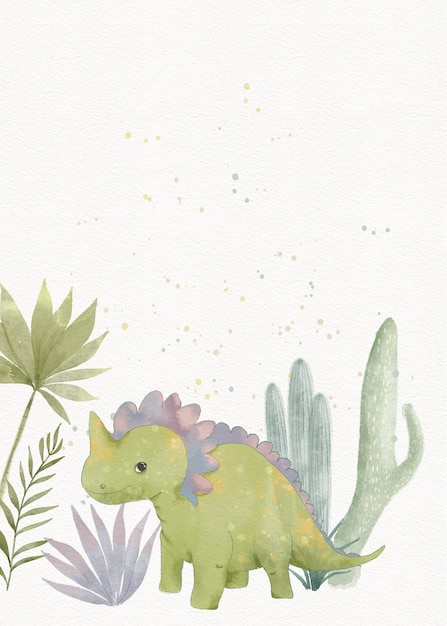This rectangular cartoon image features a whimsical, dinosaur-themed wallpaper design. Set against an off-white, light stone-colored background, green and light gray dots are scattered across the top portion. 

In the lower section of the image, a variety of plants create a lively scene. On the left, two green plants stand out: one with a tall stalk and fan-shaped oval leaves at the top, and another with a stem and leaves dispersed along its length. Additional cactus-like shapes are present on both the left and right side of the scene. A distinct purple plant adds a splash of color to the ground area on the right.

Dominating the center of the image is an adorably stylized green Stegosaurus-like creature. This dinosaur has a small horn on its snout and is facing left. Its body is adorned with purple ridges that extend from behind its head all the way to its tail, contributing to its charming appearance.